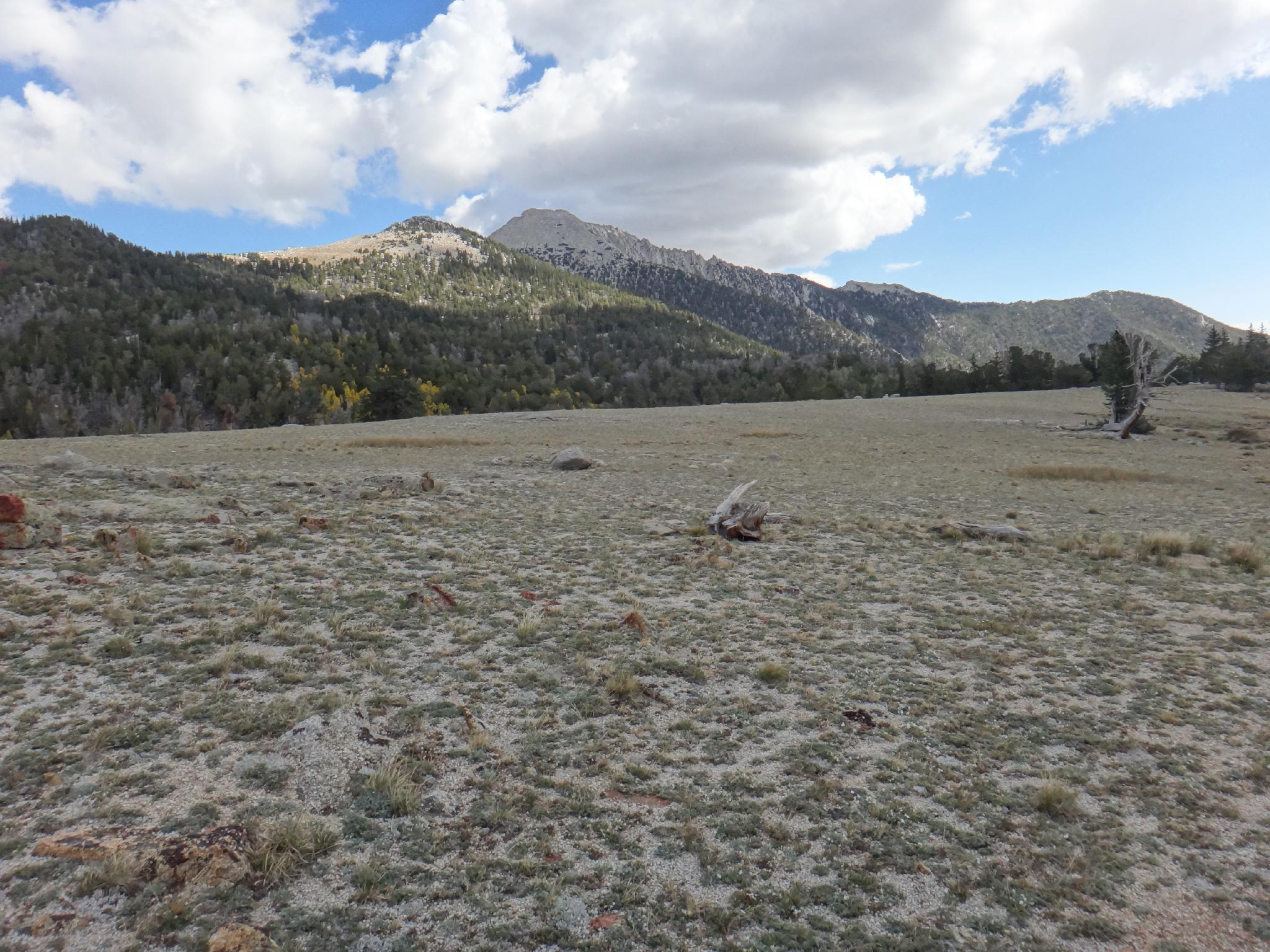The photograph, taken from a low angle, captures a dry, barren prairie landscape. The foreground is characterized by sparse, scrubby vegetation and patches of light brown dirt interspersed with rocks and pieces of wood. A prominent animal skull, possibly a cow's, rests at the center of the image, underscoring the harshness of the environment. To the right, a barren tree stands solitary and stark. The background features large hills and mountains adorned with lush green pine trees, although their summits are barren of vegetation. The sky above is a brilliant blue, dotted with fluffy white clouds, with sunlight illuminating one of the hills' peaks. The overall scene evokes the rugged beauty of a desolate region, potentially set in the northwestern United States, such as Montana, Wyoming, North Dakota, or Idaho.